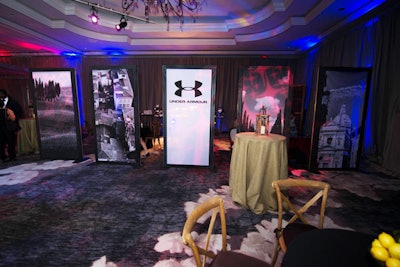The image captures a well-decorated room, possibly a backstage area or a venue preparing for an event or awards ceremony. Dominating the scene is a large, tall poster bearing the Under Armour logo, prominently displayed against a light background. Accompanying the main poster are several other smaller advertisements or artworks, some depicting landscapes and abstract designs. The room features multicolored fluorescent lighting on the ceiling, casting blue and pink hues across the space. A high-top table draped in a light green or beige tablecloth, likely intended for cocktail conversations, is notable in the foreground. There are also a couple of chairs present, set against a dark gray carpet. The overall lighting includes spotlights, enhancing specific areas of the room, and no people are visible, emphasizing the room’s setup and decor.